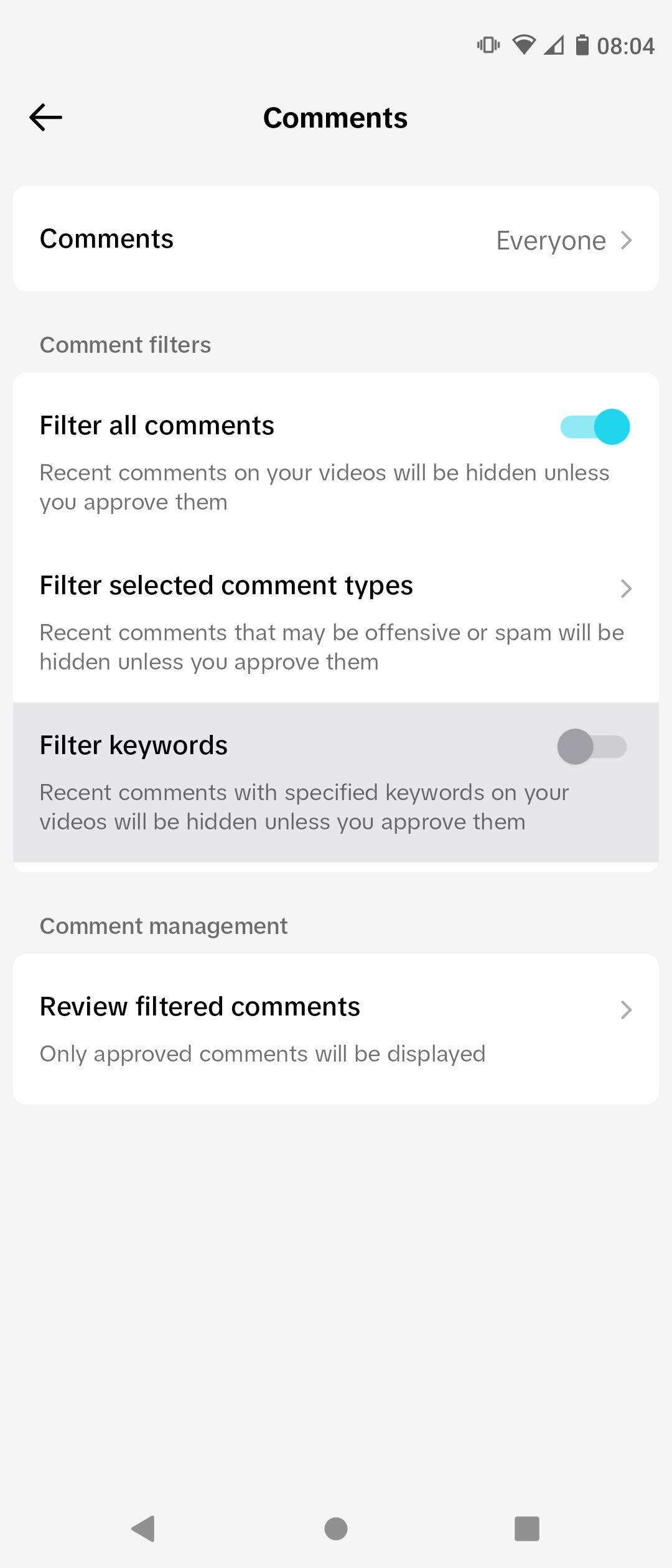The image shows a smartphone screen displaying the 'Comments' section of a social media or video-sharing app. The time at the top reads 08:04. At the uppermost section, there's an arrow pointing to the right next to the word "Everyone," indicating a navigation option. A bright turquoise 'Filter All Comments' button is turned on, highlighting that recent comments on the user's videos will be hidden unless approved.

Below this, there is a detailed explanation: "Filter Selected Comment Types - Recent comments that may be offensive or spam will be hidden unless you approve them." An arrow suggests further options to view those filtered comments. The next section titled "Filtered Keywords" indicates that recent comments containing specific keywords will be hidden unless approved, but this filter has not been activated.

Further down, a "Comment Management" heading appears, with the text "Review Filtered Comments - Only approved comments will be displayed," reinforcing the idea that the user is reviewing their comment moderation settings. The overall scene depicts a user navigating and adjusting their comment filters and management options on their smartphone.